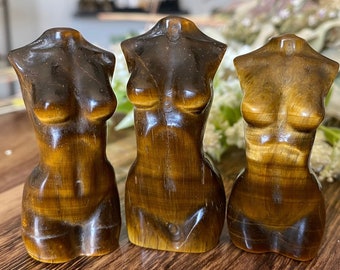In this small, square photograph, we observe three intricately carved gemstone bust sculptures of women's torsos, crafted from tiger eye gemstone. Each sculpture prominently features the chest, midriff, and upper thighs, but lacks arms and heads, terminating abruptly at the neck and upper thigh regions. All three statues share a similar slim build and are positioned side by side on a polished wooden table, which showcases a dark, lustrous grain running upwards to the right.

The tiger eye material of the sculptures exhibits a rich, amber hue with distinctive yellow-brown striations, contributing to their striking appearance. The sculpture in the center appears slightly taller compared to the ones positioned on either side. Additionally, the lighting plays a role in their coloring; the sculpture on the right has a lighter top and darker lower section, whereas the other two have the opposite gradient, being darker on top and lighter below.

In the softly blurred background, discernible elements include a cluster of white flowers and green leaves positioned on the table's right side, adding a touch of natural elegance to the scene. The rest of the background remains out of focus, providing minimal context to the setting but directing attention to the exquisite gemstone sculptures in the foreground.